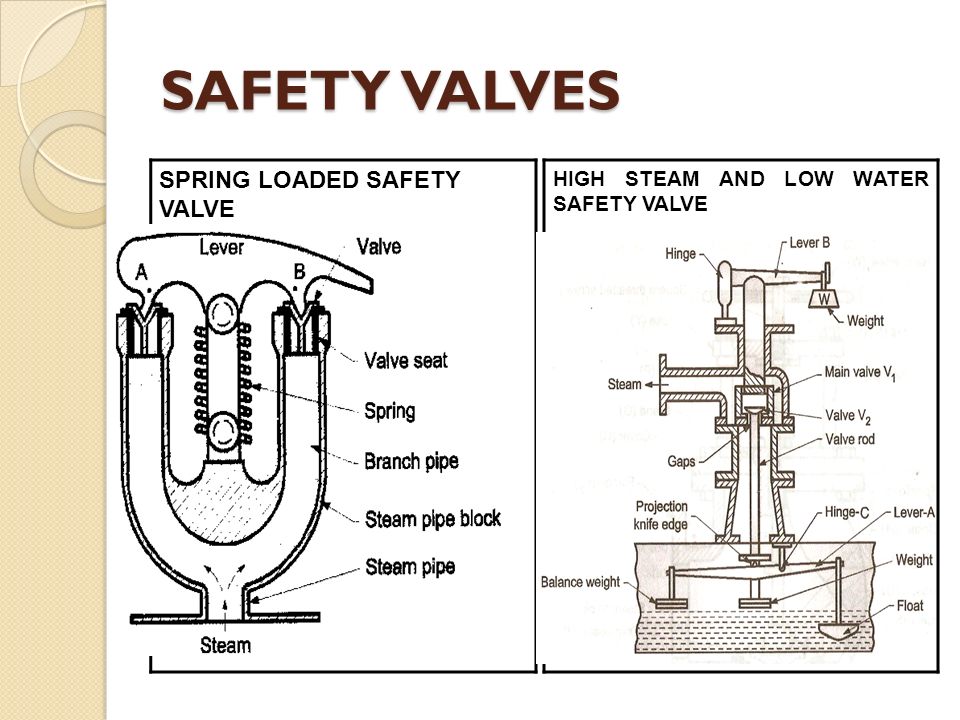The image features two detailed diagrams of safety valves, prominently labeled at the top in uppercase brown letters as "SAFETY VALVES." The left diagram depicts a spring-loaded safety valve, distinguished by its U-shape and a darker color compared to the right diagram. This spring-loaded safety valve consists of a lever at the top and includes multiple labels identifying its parts. The components are detailed as follows: the upper section features a lever attached to a valve positioned on the top right of the U-shape, which further includes a valve seat. Within the U-shape, there is a spring situated between the labeled branch pipe, with the outer layer marked as the steam pipe block and the bottom identified as the steam pipe. Additionally, steam is depicted as rising upward within the U-shape.

The right diagram illustrates a high steam and low water safety valve, featuring numerous labels that detail its components, but appears visually less complex than the left valve. This diagram incorporates variations in coloring, with a notable lighter hue, and is identified with its respective label "HIGH STEAM AND LOW WATER SAFETY VALVE." Overall, the comparative simplicity of the spring-loaded valve on the left contrasts with the complexity and multiple labels of the high steam and low water safety valve on the right, both clearly illustrated to provide a comprehensive understanding of their structure and function.